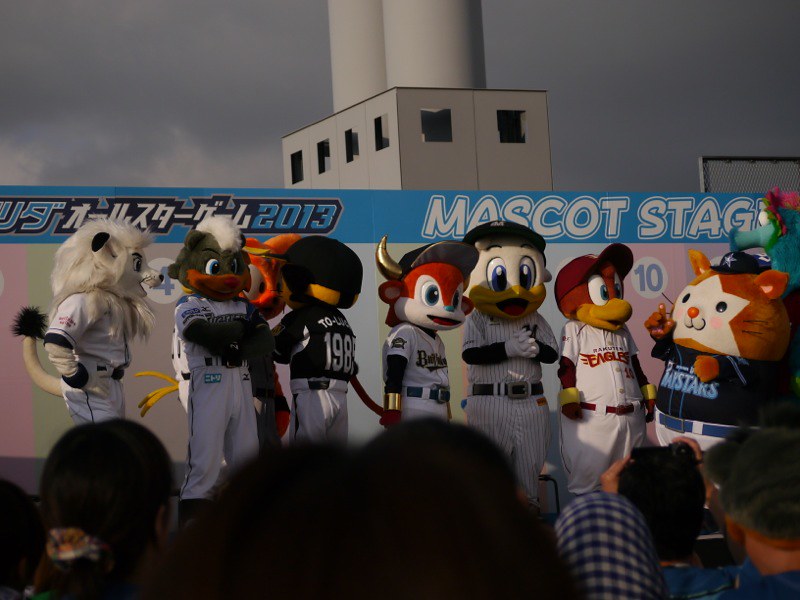This color photograph, taken outdoors in 2013, captures a lively scene on a stage labeled "Mascot Stage." Set against a backdrop of a gray, overcast sky and a building with six black windows, the stage features a lineup of seven to eight colorful mascots, each dressed in baseball uniforms. The mascots represent various animals, including a fox, birds, a chipmunk, a lion, and a notably rotund cat positioned on the right. Japanese text is visible, suggesting that the event takes place in Japan. In the foreground, the blurry heads of numerous spectators can be seen, capturing the moment with their cameras.